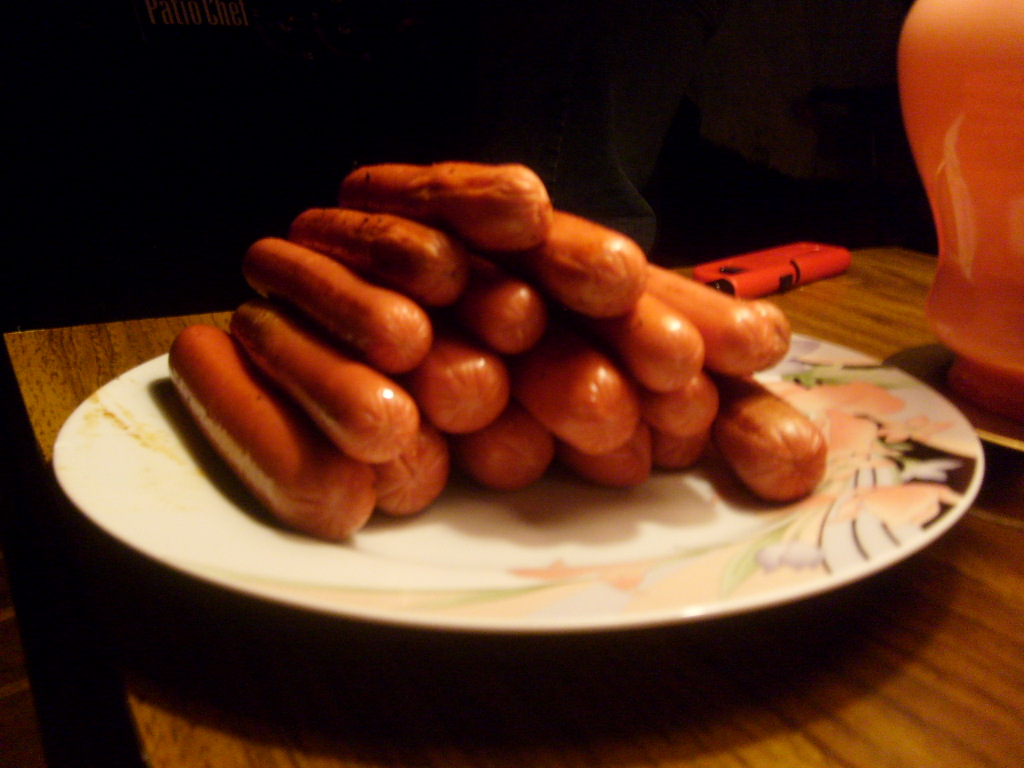The image depicts a white circular plate with a floral pattern on the right side, featuring shades of light pink, black, and dark green. The plate rests on a light brown wooden table, which appears to be a wood-grained countertop or an end table. The plate is stacked with approximately 15 hot dogs, arranged in a pyramid shape with six at the base, followed by decreasing rows of four, three, two, and finally one on the top. The hot dogs are light brown and have varying degrees of doneness, with some showing light grill marks while others appear more well-cooked and shriveled. In the top right corner of the image, an orange gas lighter is visible, and to the far right, part of an orange lamp or vase can be seen, adding a pinkish-orange reflection. The background is dark, providing a stark contrast to the focal elements.